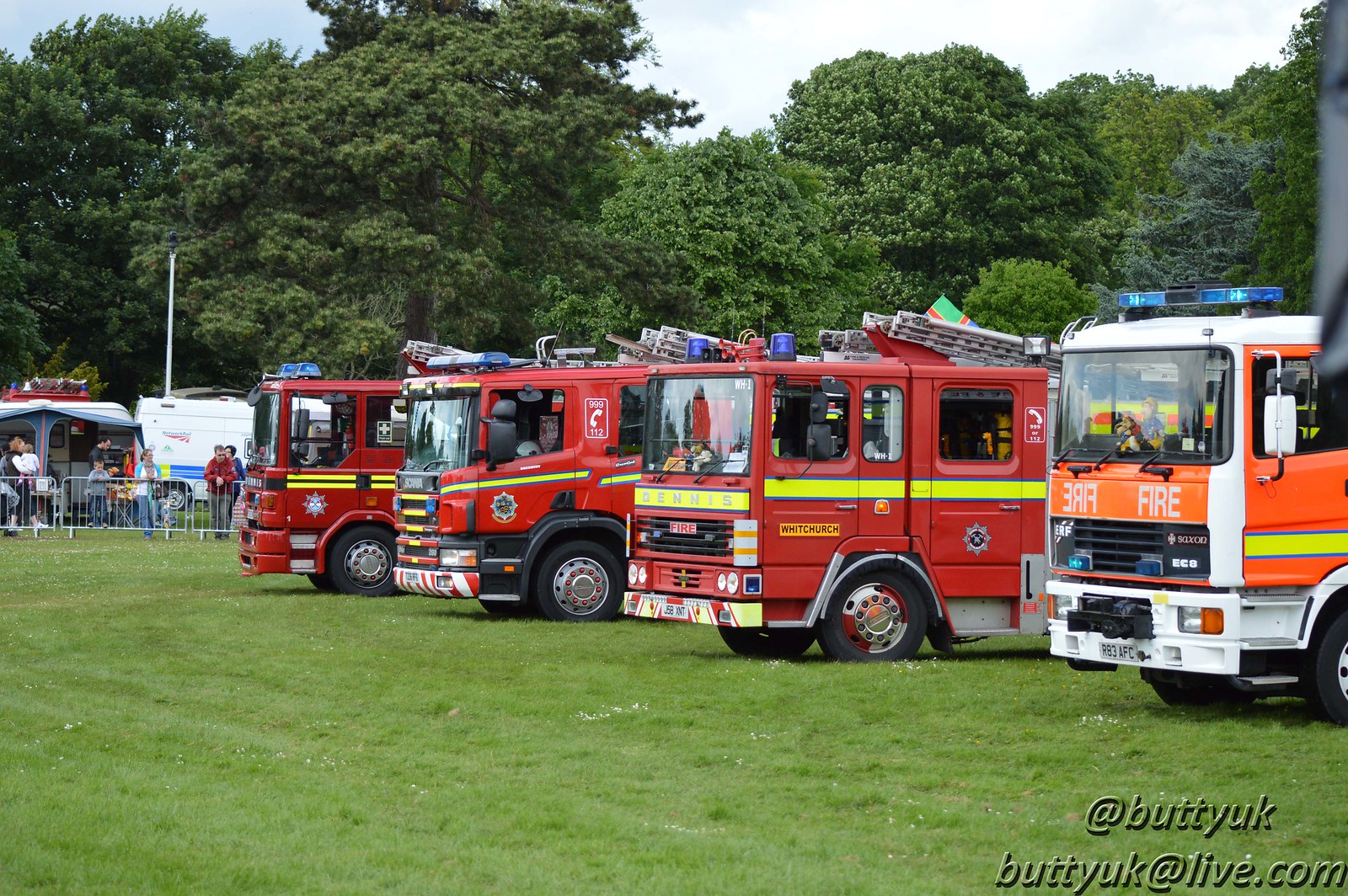In this horizontal, color photograph, four fire trucks are prominently displayed, parked in a grassy area surrounded by tall, mature trees with lush green leaves. Three of the fire trucks are painted bright red with neon yellow safety striping, while the fourth truck, positioned at the far right, is white with orange doors. The orange truck features the word "FIRE" written in large, white capital letters below the windshield, alongside a mirrored version of the word. Blue sirens are mounted on the roofs of all four fire trucks, and parts of the ladders are visible protruding from the tops.

The trucks are aligned side by side, with their noses seemingly pointing to the right, though it is suggested that the orientation of the trucks might vary. Toward the left side of the photograph, there is a metal railing and a fenced-off area where several people are gathered. Among them, a person in a red sweatshirt stands out. The backdrop includes some indistinct vehicles, possibly campers, indicating that the setting might be a campground, county fair, or a festival. The scene is capped with a partly cloudy sky, showing patches of blue and an overlay of white clouds. An inscription at the lower right corner reads "@BUTTUK" with the same text repeated below, followed by what appears to be an email address, potentially "@live.com."